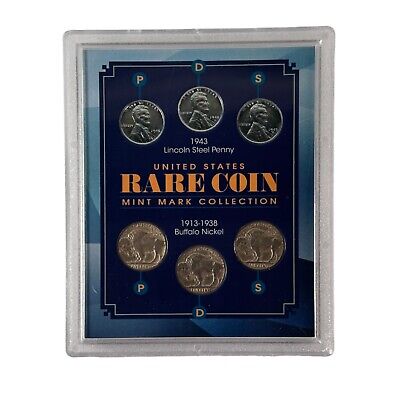This photograph showcases a carefully packaged coin collection within a sealed plastic display case. The case features a blue background with a varying shades blue border. At the center of the display, bold orange text states "Rare Coin," highlighting the set's uniqueness. The collection is titled "Mint Mark Collection" and prominently features "1943 Lincoln Steel Penny, United States" at the top and "1913-1938 Buffalo Nickel" at the bottom.

The top section of the display houses three 1943 Lincoln Steel Pennies, arranged in a row. Each coin is marked above with a letter encircled: P, D, and S. These coins are distinctly steel-colored, giving them a silver appearance. The bottom section holds three 1913-1938 Buffalo Nickels, arranged similarly with corresponding mint marks below as P, D, and S, which have a coppery-tin hue. The overall layout of the coins forms a hexagonal shape within the display case, presenting a visually appealing arrangement.